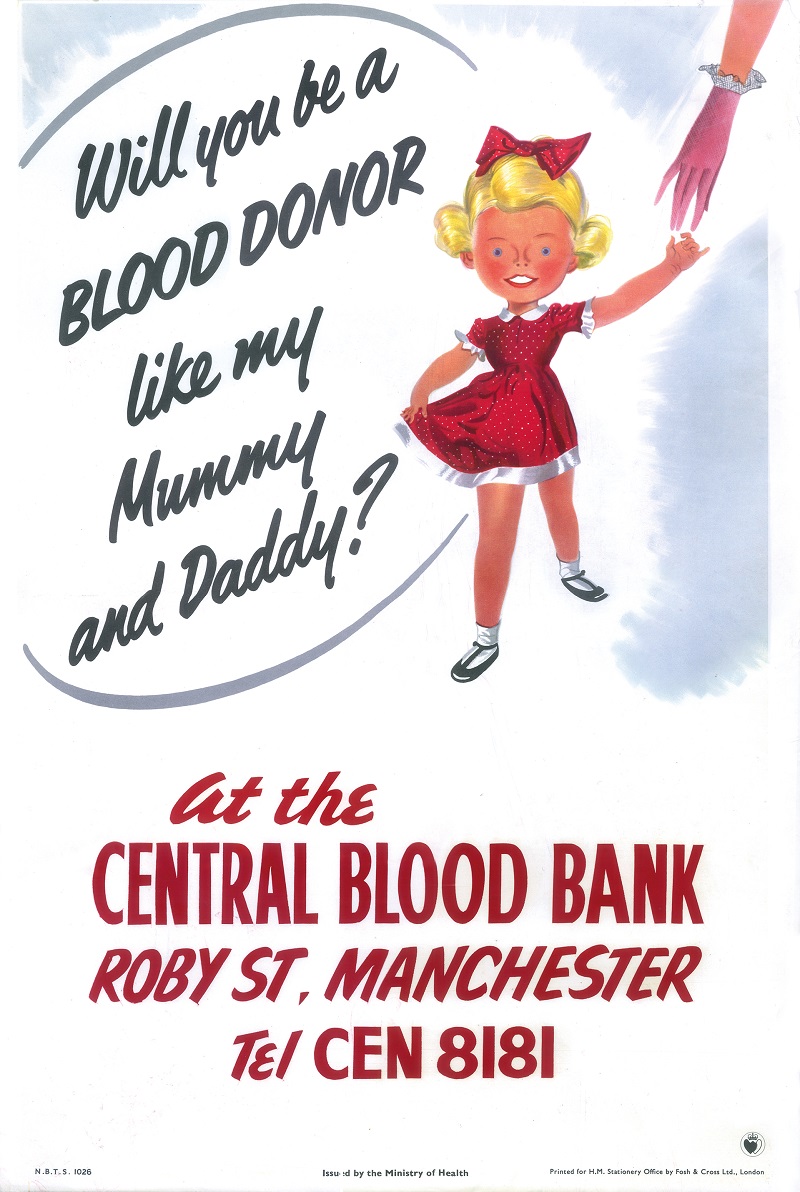This vintage-style graphic advertisement for blood donation features a detailed illustration designed to evoke a nostalgic feel. At the center of the image is a little blonde girl, clad in a red polka dot dress with white trimmings, finished with a matching bow on her head. Her outfit includes black shoes and the dress, which has short sleeves extending slightly beyond her shoulders and a hemline that ends mid-thigh. Beside this charming figure, a feminine hand reaches out, suggesting a comforting grasp. 

Adjacent to the girl on the left, there are five lines of black text that read, "Will you be a blood donor like my mommy and daddy?" This text is prominently positioned against a white background. Below this, in red text, is a paragraph providing the details of the blood bank's location: "At the Central Blood Bank, Roby Street, Manchester." The telephone contact is listed beneath this: "Tel: CEN-8181." This lovingly crafted advertisement combines the innocence of childhood with an earnest plea for blood donation, effectively utilizing a vintage aesthetic to convey its message.